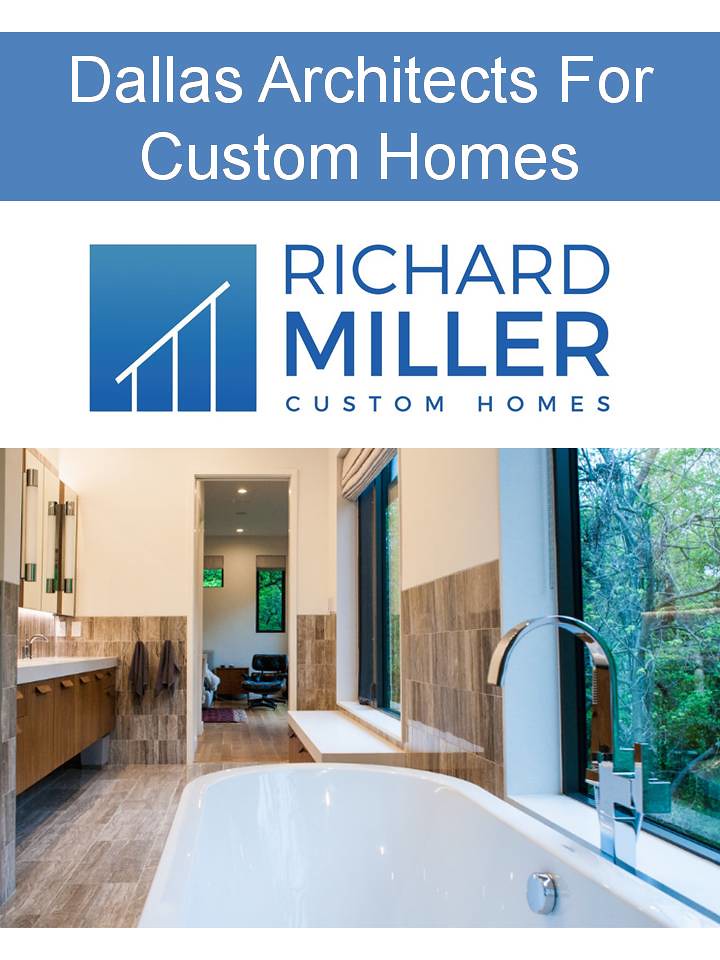The advertisement features a striking blue banner at the top with the text "Dallas Architects for Custom Homes" displayed in crisp white letters. Beneath this, the background transitions to white, showcasing blue text and a corresponding blue logo. On the left side, a square emblem resembling a partial outline of a house adds a visual touch. Adjacent to this, bold text reads "Richard Miller Custom Homes."

Below the textual details, the ad transitions to an inviting scene of a sophisticated bathroom. The floor boasts intricately tiled patterns mimicking a rich, wooden texture. Central to the image is a sleek bathtub with a unique, flat chrome faucet head, exuding modern elegance. The serene setting is further enhanced by two expansive windows, providing a captivating view of dense woodland outside.

On the left side of the bathroom, a refined counter with a polished sink is accompanied by two sizable mirrors, reflecting the room's grandeur. Additionally, a doorway offers a glimpse into an adjoining space, where a chair is visible, hinting at a connected living room, bedroom, or family room, creating a seamless blend of luxury and comfort.